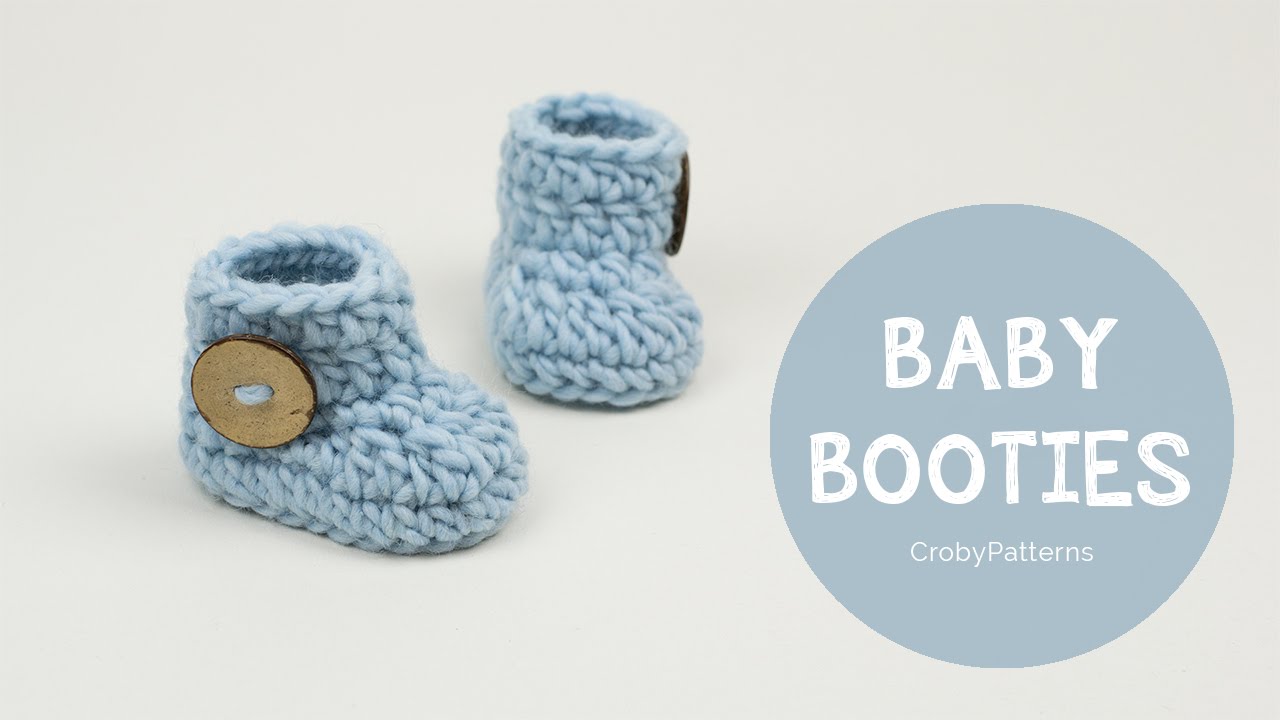The image features a pair of small, hand-knitted baby booties crafted from light blue yarn, each adorned with a brown wooden button on the side. Positioned at an angle, one bootie displays its side detail with the button prominently visible, while the other points slightly forward, allowing a view of the button's outline. The background is predominantly white, enhancing the clarity of the booties. To the right of the booties, the image includes a round, darker blue circle with the words "Baby Booties" in white lettering, and just below this, "Kroby Patterns" appears in smaller white text, suggesting this image serves as an advertisement. The overall aesthetic maintains a soft blue and white color scheme, creating a serene and inviting visual experience.